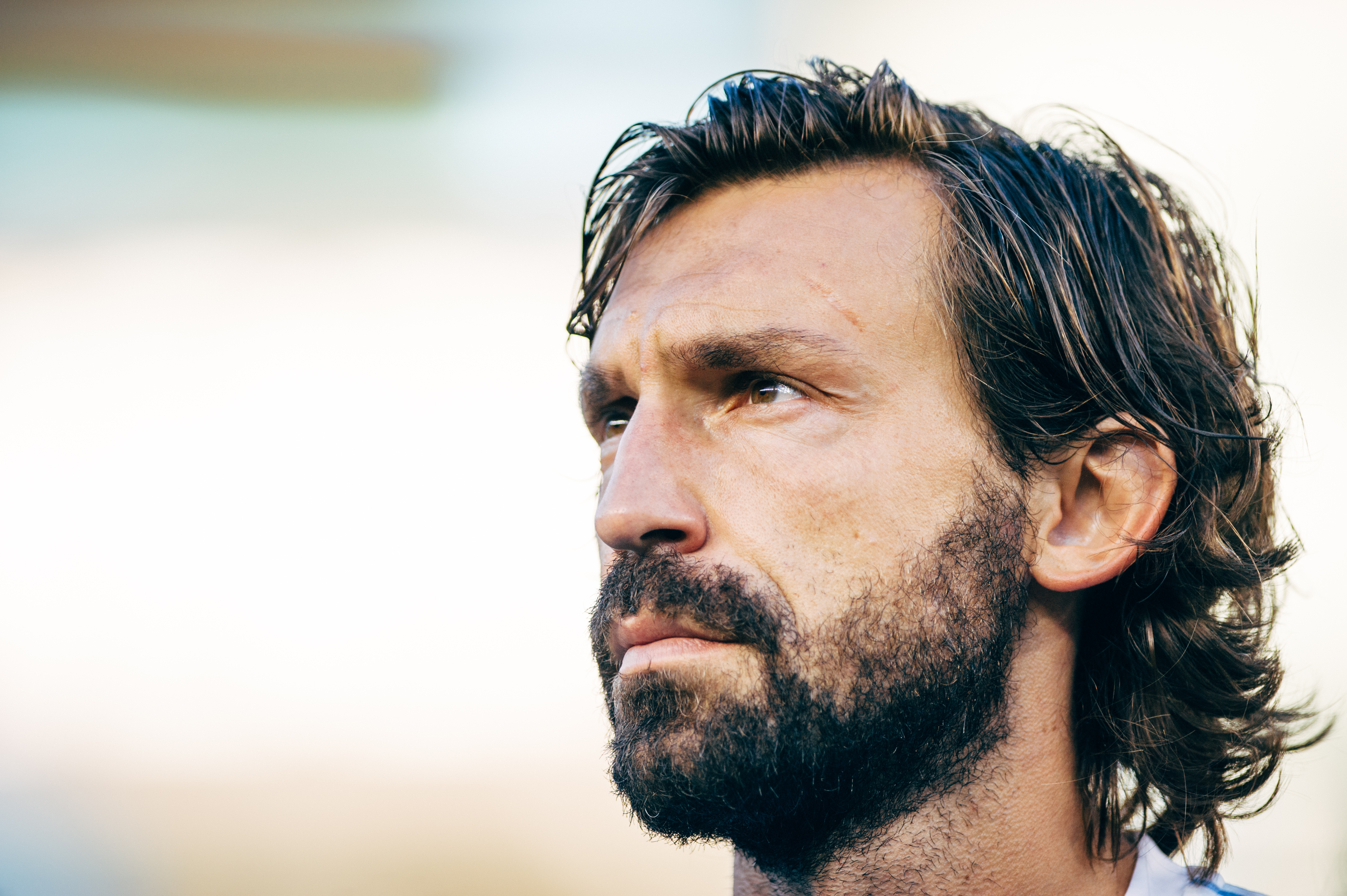The photo features a defiant-looking young man with almost shoulder-length wavy hair that appears slightly greasy, with light brown and blonde interspersed highlights. His hair is parted near his left temple and swoops up slightly in the front. He has a thinnish black mustache and a somewhat thin beard that lightens near his earlobe and chin. His facial expression is serious as he gazes intently to the upper left. He has brown eyes, not very bushy eyebrows, and an ordinary nose. His olive-tanned skin is all that stands out against the blurred, sharp white background, and a tiny bit of his whitish-blue shirt is visible near the collar. The entire composition directs attention to his contemplative and focused demeanor, although it is unclear what he is looking at.